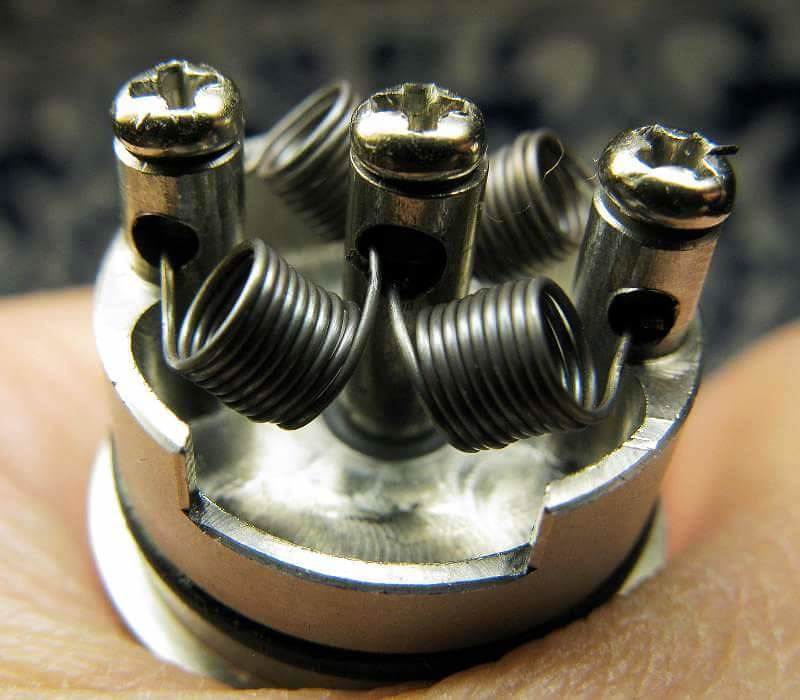In this detailed photograph, a round, silver metallic piece is prominently displayed, held in the palm of a hand with light skin. The image, though slightly blurry in the background, focuses on the intricate details of the object. It features three cylindrical posts arranged in a row, each topped with a Phillips head screw. Beneath these posts, there are four coiled springs, two in the front and two in the back, intricately threading through large holes at the base of the cylinders. This assembly sits atop a black washer-like base, which further accentuates the metallic texture and sheen of the piece. The hand's slight wrinkles and the indentation of the skin add a subtle indication of the object's weight and the grip applied to hold it. This technological component, likely part of an electrical appliance, showcases precision-engineered fasteners and coils, integral to its function.